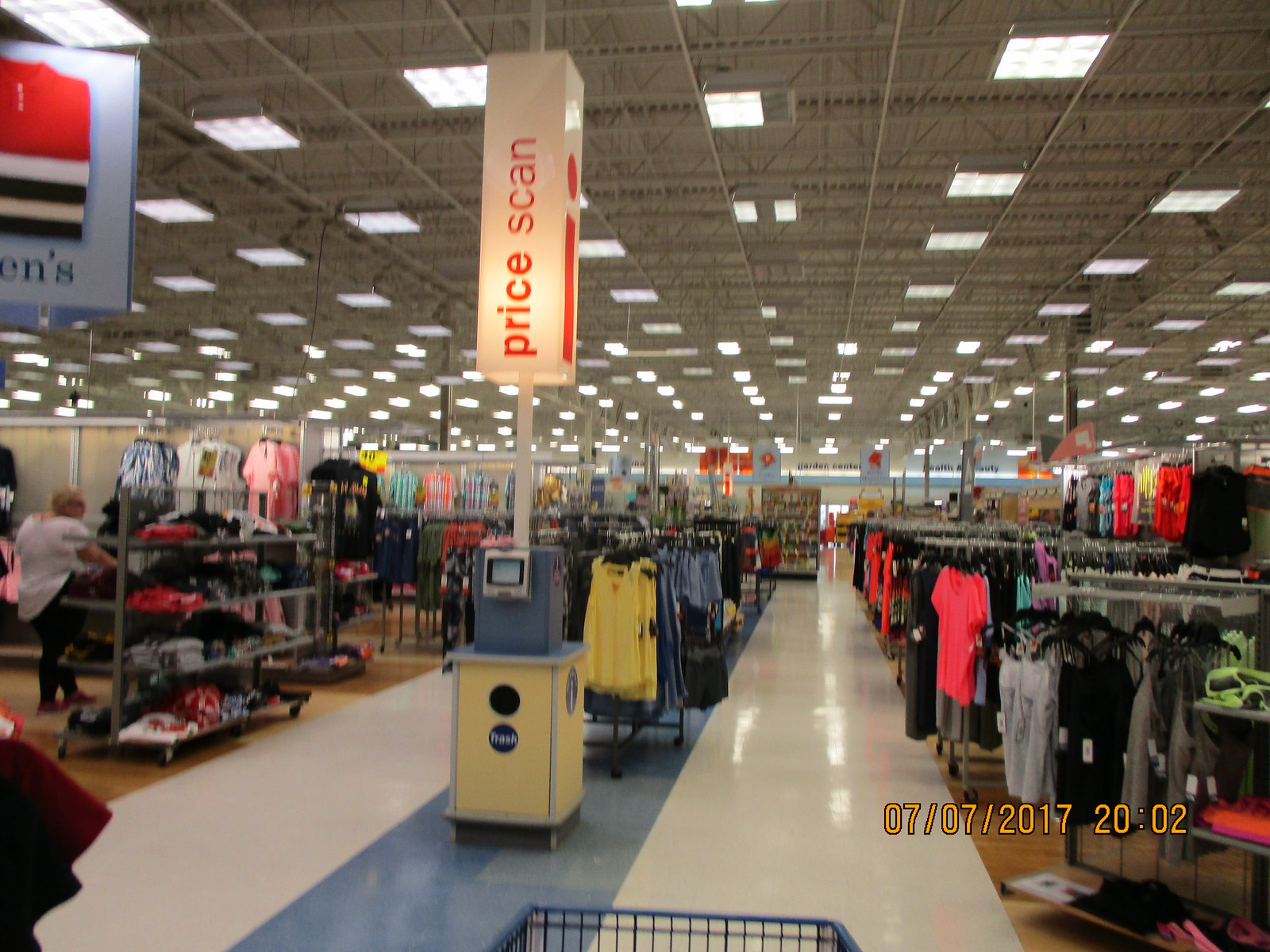The photograph captures the bustling interior of a large department store, resembling a warehouse with its open, industrial-style white ceiling adorned with square fluorescent lights. The expansive space is filled with neatly arranged aisles showcasing a plethora of clothing and garments. The edge of a shopping cart, being pushed by the photographer, is visible in the foreground, adding a sense of immediacy and perspective to the scene. Shelves brimming with meticulously folded clothes line the aisles, while racks overflowing with hanging apparel create a tapestry of textures and colors. A price scanner is prominently positioned in the center aisle, offering convenience to shoppers. The image is time-stamped 07-07-2017, 20:02, indicating it was captured in the evening.